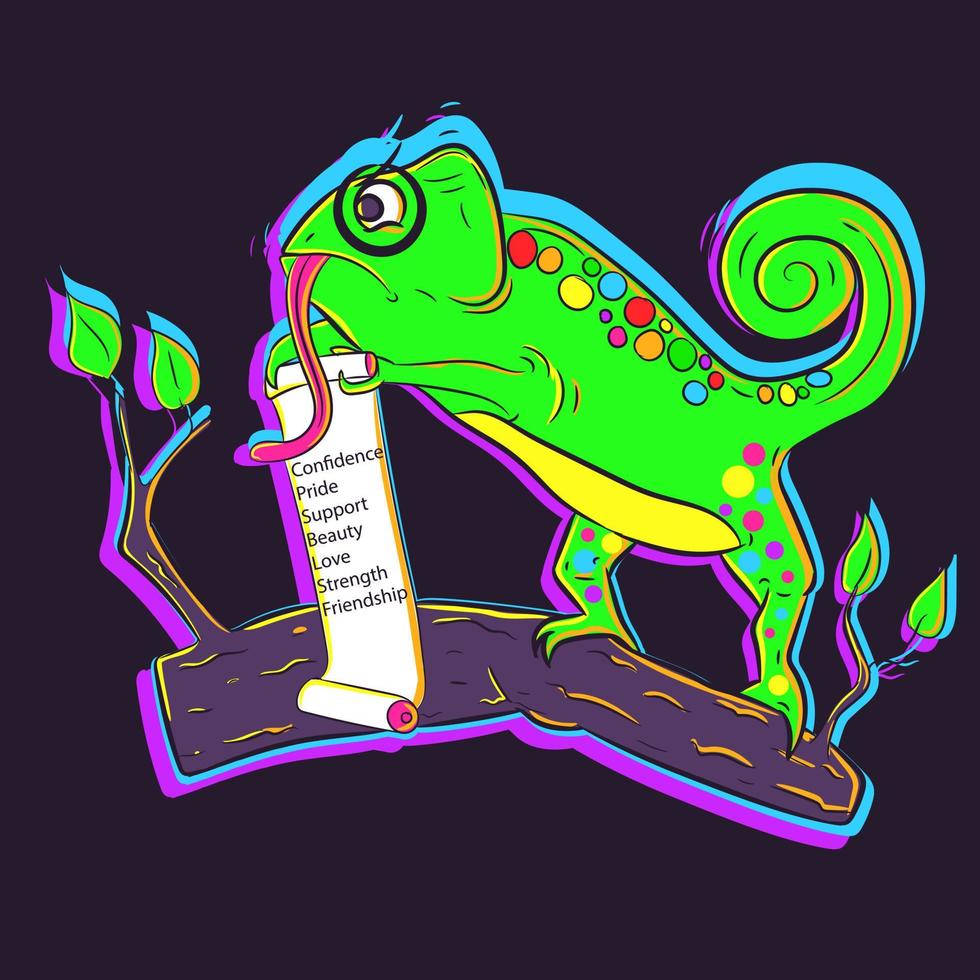This is a digital cartoon image featuring a vibrant, neon green chameleon perched on a purple tree branch adorned with green leaves. The chameleon's skin showcases a variety of colorful spots, including red, orange, yellow, blue, pink, and purple, which extend onto its legs. A striking pink tongue extends from its mouth, illustrating its focus. The chameleon is holding a green scroll with both front limbs, and in black text, the words "Confidence, Pride, Support, Beauty, Love, Strength, Friendship" are inscribed on the scroll. Notably, the chameleon also sports a spectacle over one eye and has a violet tail. The background of the image is a deep purple, enhancing the vibrancy of the chameleon and its surroundings.